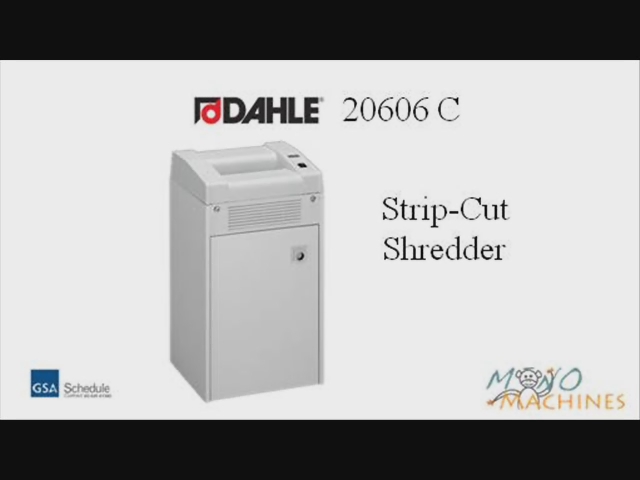This photograph is an advertisement for the DAHLE 20606C Strip Cut Shredder. The image features a vertically positioned, off-white paper shredder prominently centered against a solid white gradient background, bordered by black strips at the top and bottom. The shredder, which appears to be of moderate height, includes a front compartment door used to access the shredded paper container. The door, which occupies most of the front surface, is equipped with a vent and appears to have a key lock option. The machine has a top slot for easy paper insertion and only a few controls, emphasizing its simple and minimalist design. Centered at the top of the image, the model number "DAHLE 20606C" and the label "Strip Cut Shredder" are prominently displayed. In the bottom right corner, the logo and name "Mono Machines" along with a monkey graphic are visible, while the bottom left corner carries the initials "GSA SCHEDULE."